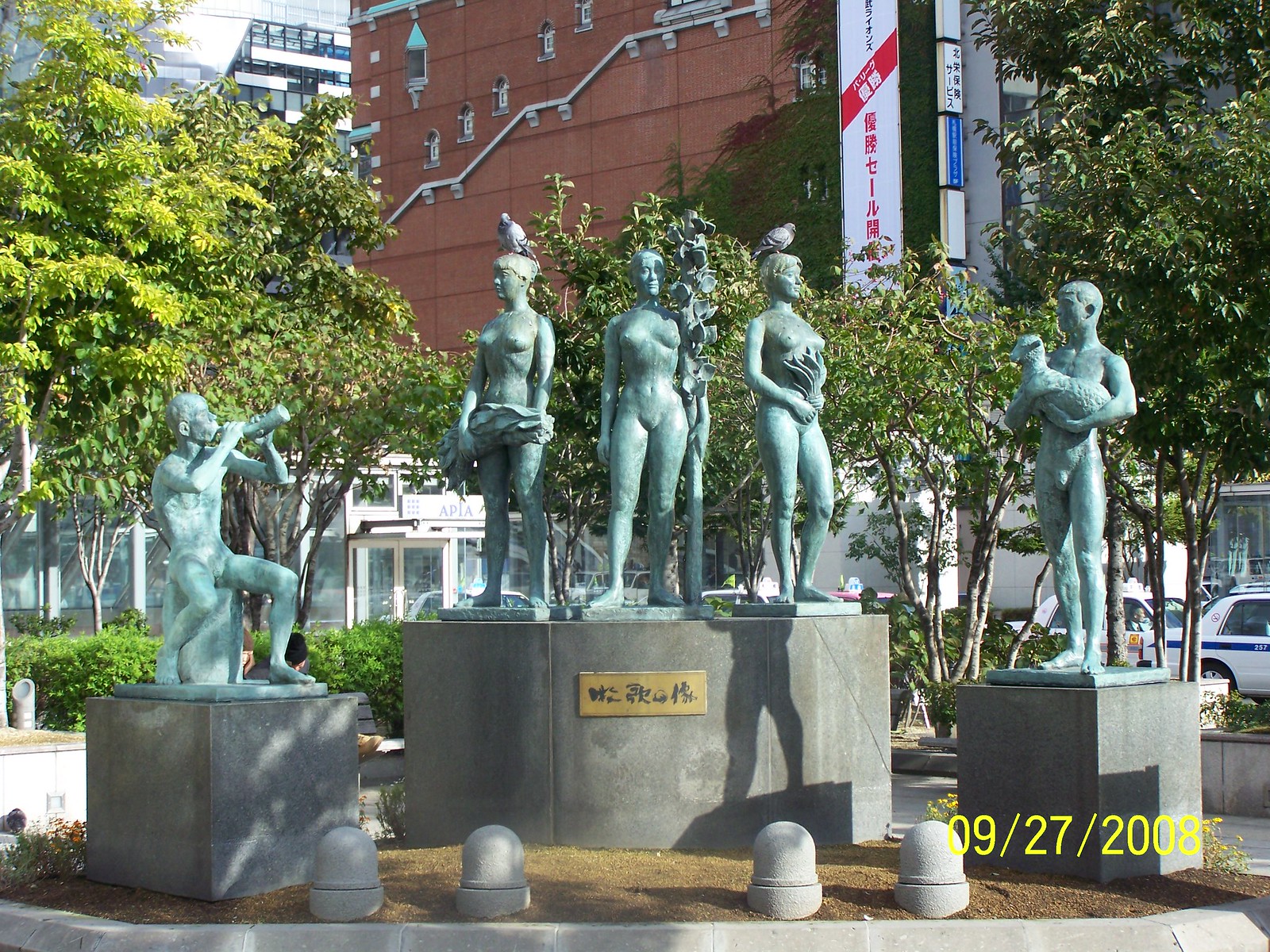This is a detailed outdoor photograph taken on a sunny day, dated 09/27/2008, as indicated by a yellow date stamp in the bottom right corner. The image features a group of five statues placed on three cement bases arranged in a somewhat circular concrete area. The central base is round and taller than the two square bases on either side. The statues exhibit a green patina, giving them a teal greenish-gray color.

The central, round base supports three statues of women. The figure in the middle holds a staff in her left arm and gazes slightly to the right. The woman on the left cradles what appears to be plants in both arms, looking slightly to the left. The woman on the right has wavy hair, cascading upward, and holds a wavy object.

On the left square base sits a man playing a horn-like instrument while on the right square base, another man stands holding a sheep, looking to the left. Both male statues are nearly nude, contributing to the shared theme of minimal clothing among all the statues.

Notably, live birds, likely pigeons, are perched atop the heads of the two outermost female statues positioned on the central base. In the background, there are green leafy trees and a large red brick building. Additionally, signs with Asian characters suggest the photograph might have been taken in an Asian country. The scene is well-lit, casting noticeable shadows around the statues.